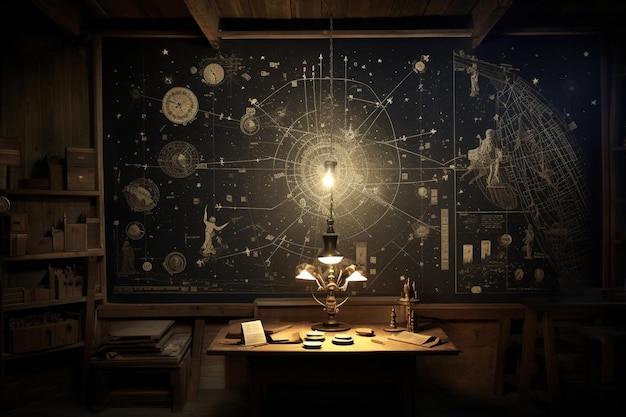The image captures an intricately detailed scene that appears to be a blend of a home library and an artist's studio, enveloped in a warm, subdued ambiance. Dominating the scene is a expansive, artistic canvas mounted on the wall, depicting celestial and astrological themes. This canvas showcases a black sky filled with stars, planets, and constellations, alongside a web of arrows and astrological symbols rendered in neutral tones of black, white, brown, and gold. Below this captivating artwork is a central desk, possibly doubling as a dining table, adorned with a few saucers, papers, and a book, suggesting a lived-in, intellectual environment. The desk features a distinctive chandelier-style lamp suspended on a long chain, casting a soft light over the workspace. Additionally, a smaller light bulb hangs halfway down into the room, enhancing the overall dim setting. To the left, there's a shelving unit with various objects, likely books and boxes, adding to the scholarly atmosphere. Seating spaces are hinted at but remain obscured by the room's low lighting, further intensifying the intimate, contemplative mood of this unique space.